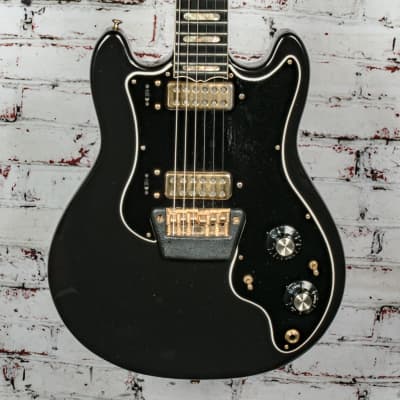The image depicts a black electric guitar hanging on a rustic white-painted brick wall with patches of red brick showing through. The guitar is prominently featured with its base in clear view, revealing its shiny black panel and light-colored strings. On the right side towards the bottom of the base, two silver dials with black bases and gold-colored knobs are visible. The guitar also has bronze-colored frets and a white stripe around its edge. Additionally, there are two switch-like buttons, likely for controlling the electronics, and a black input jack underneath them. This detailed, decorative but functional instrument is set against the textured backdrop of the partially exposed brick wall, creating a striking visual contrast.